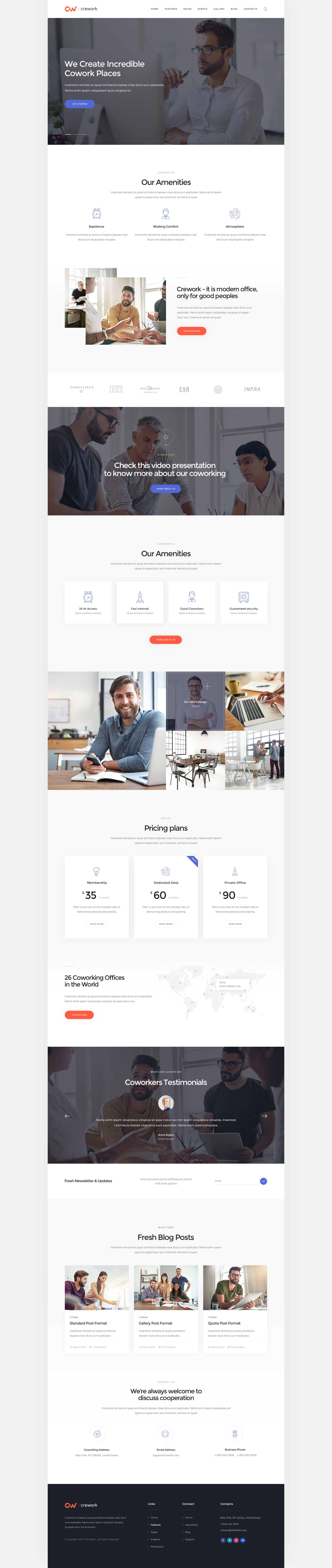A graphical depiction of an extensive webpage predominantly in white. The webpage features various graphics and sections that are difficult to discern due to the distant perspective. At the top, there's a photograph of a man with glasses, a black beard, and black hair, seated at a desk with a computer screen. Above him, a banner reads, "We create incredible co-work places." Below this, a group of people are seen smiling and sitting together around a communal area, accompanied by an orange button. Further down, another group of men is featured next to a blue button with the text, "Check this video presentation to know about our co-working." Additionally, there are sections with two men and a woman, interspersed with more orange buttons and blue banners. The pricing information is visible, listing three tiers: $35, $60, and $90.